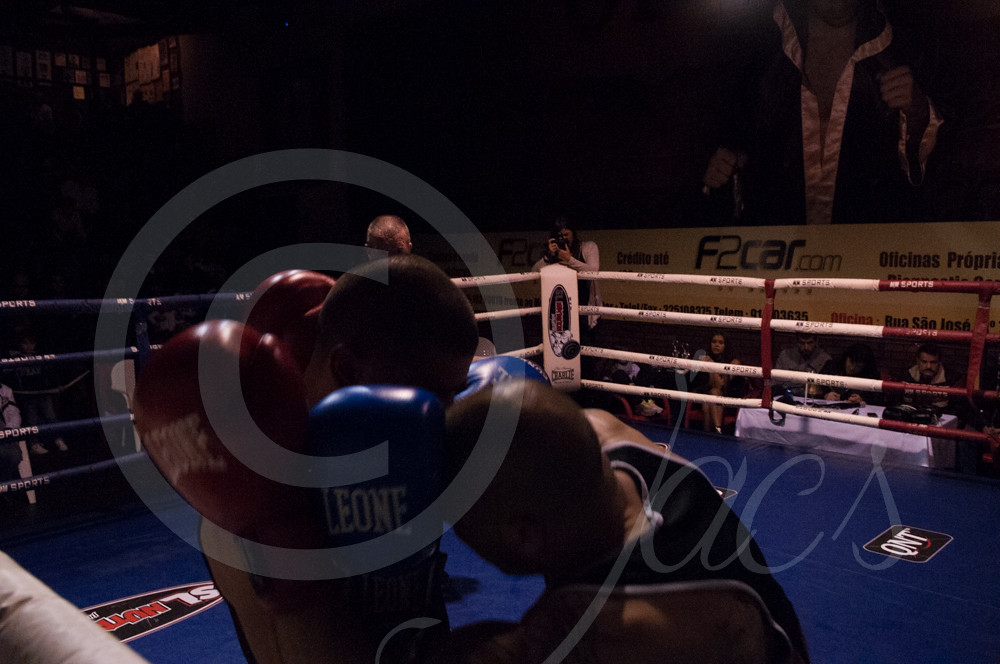This is a color photograph capturing an action-packed moment during a boxing match in a dark, dimly lit arena. In the foreground, two boxers are engaged intensely, one with blue gloves and the other with red gloves, both branded 'LEONE'. The boxer in darker blue appears to have his arm around the boxer with the blue gloves, while the one with red gloves has his arm over his opponent. The scene is partially obstructed by a large copyright watermark featuring a circled 'C' and the text 'J-A-C-S'. The boxing ring features a blue floor mat with scattered lettering, including 'Q' and 'T', and ropes colored red and white on one side and blue and white on the other. In the background, the top of the referee's head and a photographer with a camera are visible, alongside a prominent yellow banner with 'F2Car.com'. The dark setting of the arena reveals faint outlines of spectators and additional signage around the ring, adding depth to the high-energy scene.